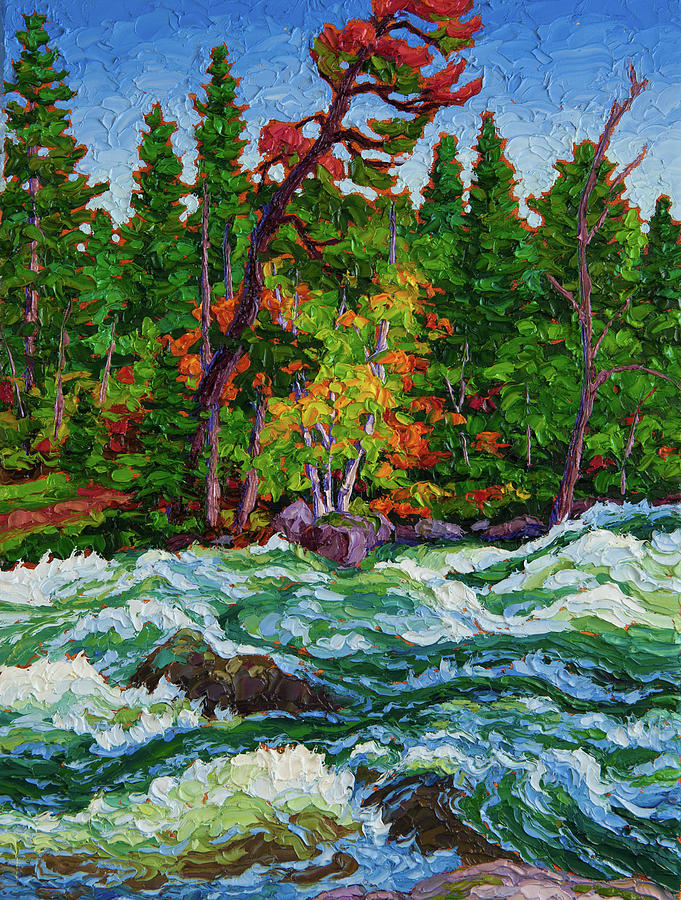This impressionist painting vividly captures a dynamic natural landscape. At the top, a textured blue sky brimming with broad, tactile brushstrokes hints at an airy atmosphere. Sprouting from the midsection, a dense forest of tall green trees stretches across the canvas, interspersed with splashes of orange, red, and brown foliage. Dominating the left third of the painting is a strikingly tall tree adorned with vibrant pink flowers, its trunk darker and more defined than the others, suggesting a lifeless grandeur as it ascends from the bottom to the top of the image. 

In the foreground, a bustling, choppy river courses through the scene, rendered in varied shades of blue with dynamic splashes of white, evoking a sense of hurried movement and turbulence. Dark rocks punctuate its flow, and waves crash violently against them, encapsulating the wild energy of the water. Along the riverbank lies a dirt path, contributing to the tactile texture of the painting. The artist's use of thick, gaudy oil paints splattered across the canvas adds to the impressionist style, creating a vivid, almost abstract representation of nature alive with motion and color.